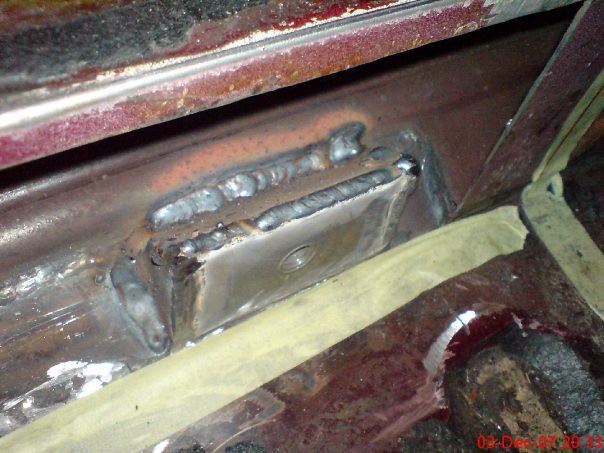The image is a detailed close-up of a heavily weathered metal object, possibly part of an old car or machinery, with extensive signs of corrosion and age. The surface is marked by a variety of colors and textures, including red, maroon, and reddish-brown areas with significant chipping and wear, revealing patches of chrome and silver underneath. A piece of aged, yellowed tape stretches diagonally from the bottom left corner towards the center, with another strip forming an angular path in the upper right. Just above the lower tape, a freshly welded metal plate is affixed to the container, showcasing gray and silver welds interspersed with yellow spots. Behind this, the metal appears severely rusted, displaying an orange wavy shape. Higher up, peeling layers of silver paint give way to sections covered in black and white specks, and additional red paint that is also chipping off. At the very bottom right corner of the rusty metal surface is a date inscribed in red: "03 December 07 20:33," which provides a timestamp for this weathered, industrial scene.